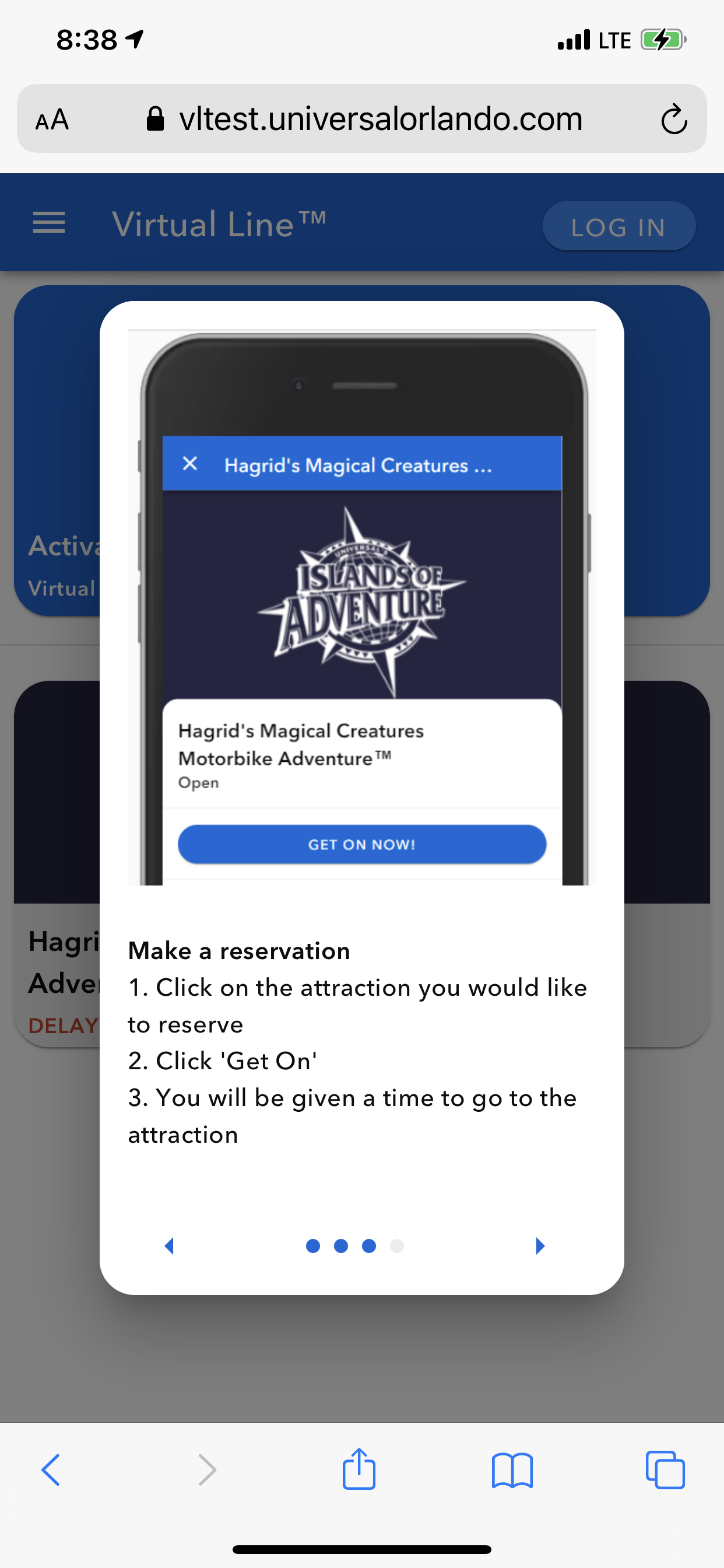A screenshot displays what appears to be a reservation interface for Universal Orlando's Virtual Line™ system, likely on an iPhone. The webpage, accessed via vltest.universalorlando.com, features a prominent floating dialogue box superimposed on top. This dialogue box presents a visual of a smartphone with a blue bar at the top, labeled "Hagrid's Magical Creatures Motorbike Adventure™," accompanied by an "X" for closing the dialogue. Below, a compass rose logo with the text "Islands of Adventure" is visible, followed by a detailed instruction box. This box explains that users can make a reservation for the "Hagrid's Magical Creatures Motorbike Adventure™" by clicking a blue "Make a Reservation" button. This system allows guests to select a specific time to visit the attraction, thus avoiding the need to wait in a physical line.

In the background, partially obscured by the floating dialogue, the main webpage features a blue top bar with a hamburger menu icon and a "Virtual Line™" label. Additionally, there is a login button visible on this top bar. Due to the overlay, the rest of the webpage's content is not fully discernible.